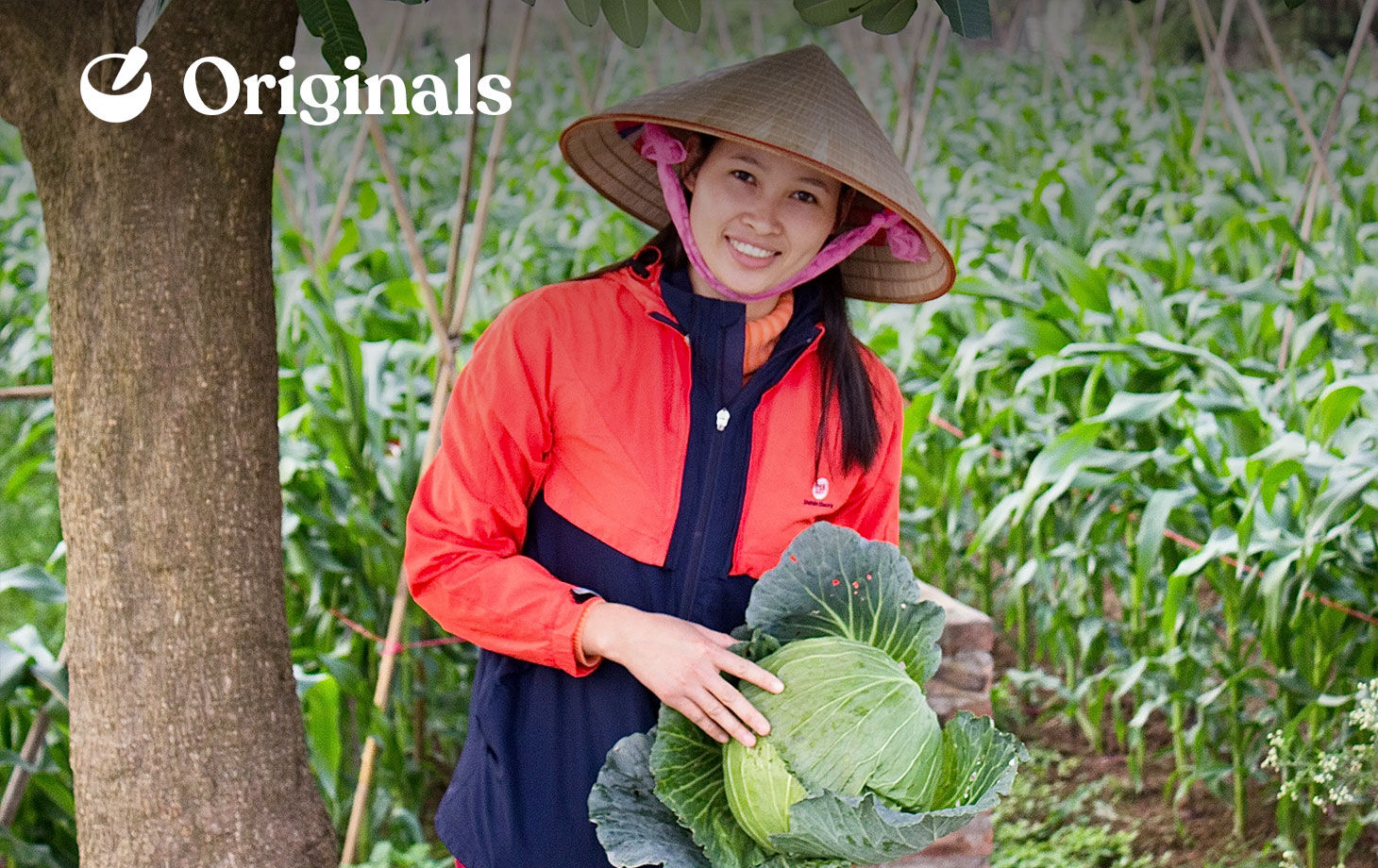In this horizontally aligned rectangular photograph, a woman of East Asian descent, appearing to be in her late 20s or early 30s, is smiling warmly at the camera. She has slightly dark skin and long, straight hair, and she is wearing a woven, cone-shaped brown hat adorned with a pink scarf tied under her chin, securing the hat. Her attire includes a striking orange and navy zippered jacket layered over an orangish turtleneck sweater. In her right hand, she proudly holds a large head of lettuce, with darker green leaves encircling the central ball of the vegetable. The background features a blurred cornfield, with tall stalks extending into the distance, and a tree trunk with fine bark visible along the left edge of the image. Adjacent to the tree is a wooden support structure with a pole extending at a steep angle. In the upper corner of the photograph, the word "originals" in bold white letters is accompanied by a small logo resembling a white bowl with a carrot. The colors in the picture are vibrant, making the scene of this beautiful harvest visually captivating.